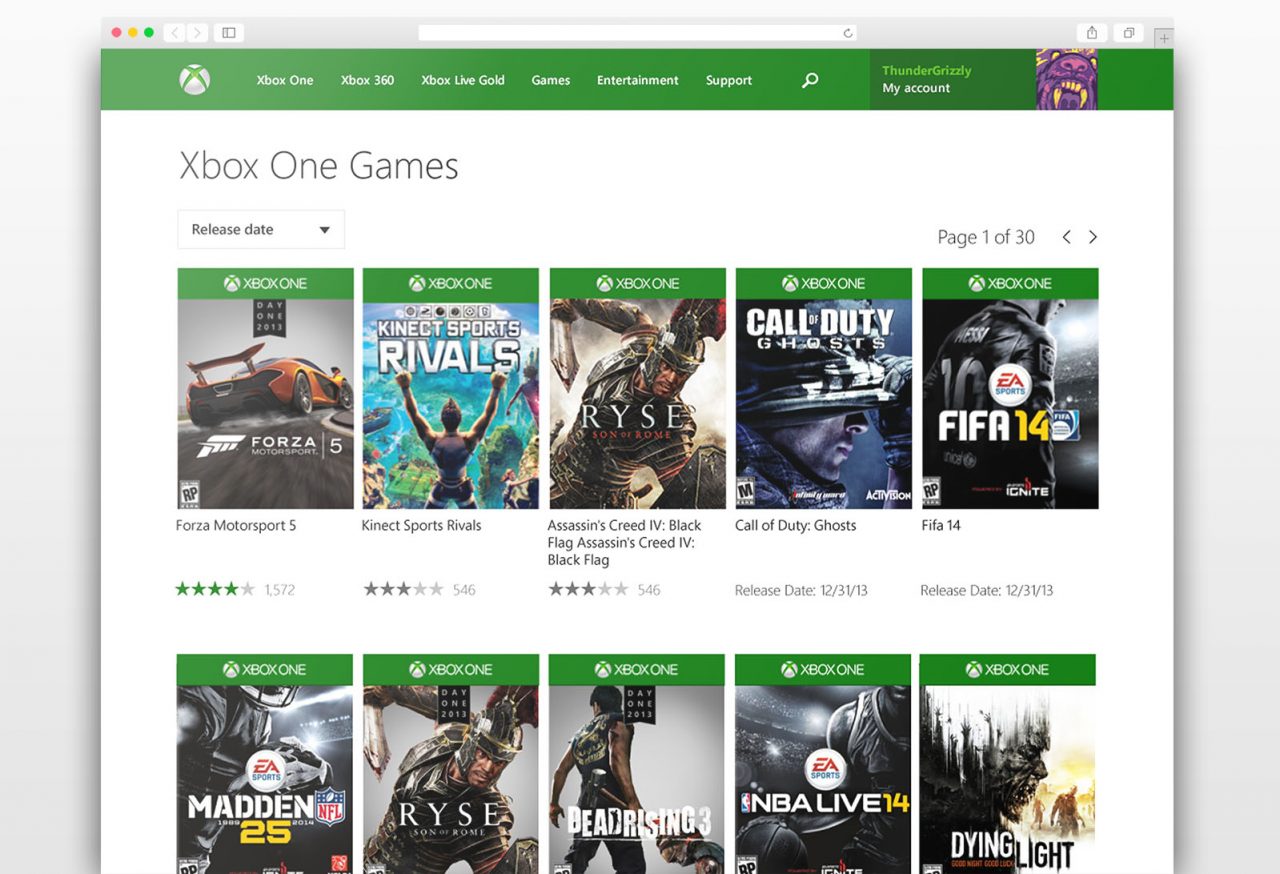This is a detailed screenshot of a browser window displaying a gaming website, overlaid on a light gray background with a medium gray shadow. The browser window features a light gray header that includes three colored circles on the top left: a red circle, a yellow circle, and a green circle. Next to these circles, there are left and right arrow buttons, followed by an icon resembling a page. At the center of the header, there's an empty URL bar with a refresh arrow on its right side. On the far right of the header, there are two light gray buttons: one with a box and an upward arrow, and another with two stacked pages.

Below the browser's header, the website's interface begins with a green header. On the left side of this header is a logo featuring a silver ball with a green X inside it. To the right of the logo, there are several navigation sections in white text: "Xbox One," "Xbox 360," "Xbox Live Gold," "Games," "Entertainment," and "Support," followed by a white magnifying glass icon. Further to the right, the header transitions to a darker green area, displaying the username "Thunder Grizzly" in green text. Underneath, in white text, it says "My Account," with a profile picture to the right showcasing a purple bear-like creature with large yellowed teeth.

The main body of the web page beneath the header is set against a white background, prominently featuring the title "Xbox One Games" at the top. Below this, there are rows of Xbox games displayed, each game likely represented by its cover art.